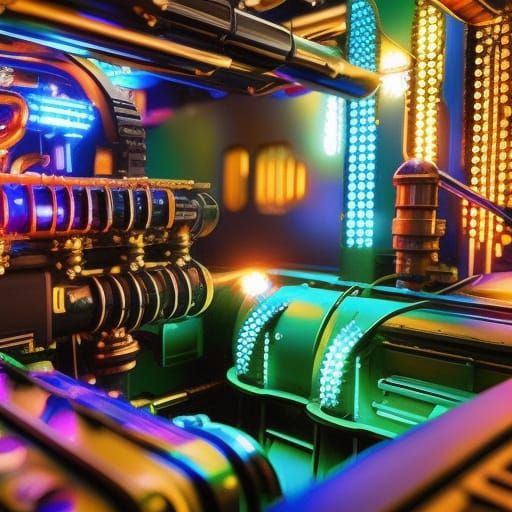This is a vibrant, computer-illustrated image, possibly a screenshot from a video game, depicting an enigmatic room filled with an array of colorful lights in green, yellow, and blue hues. The left side of the image features intricate brass machinery, adding a sense of industrial complexity. At the bottom right corner, a walkway is visible, partially obscured by the vibrant glow. The room's purpose is ambiguous, with no discernible characters, writing, plants, animals, or vehicles present. The intricate details and the harmonious play of light and color create an immersive, otherworldly atmosphere.